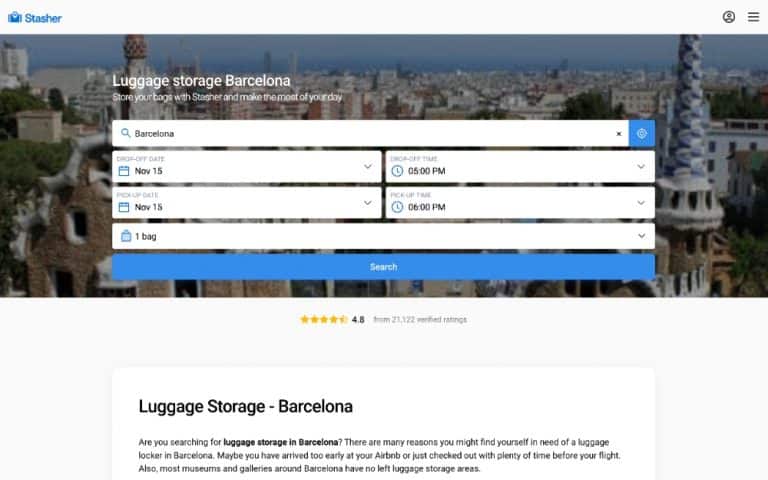This is a detailed caption for the provided image description:

---

The image displays the homepage of the Stasher website, designed for luggage storage services. In the upper left-hand corner of the screen, there is a blue briefcase icon next to the Stasher logo displayed in medium to dark blue font. On the opposite corner, the upper right-hand side, there are profile and context menu options. The main content highlights a search for luggage storage in Barcelona, with a search bar preset for a start date of November 15th at 5 p.m. and an end date of November 15th at 6 p.m., indicating a one-hour storage period for one bag.

The search bar is designed as a blue rectangle, resembling a spacebar, with white text. The background image features Barcelona, Spain. The service is highly rated, boasting an impressive 4.8 stars from 23,122 verified reviews. At the bottom of the screen, a header reading "Luggage Storage Barcelona" is prominent.

Supporting text explains the convenience of using Stasher for storing luggage in Barcelona. It addresses common scenarios such as early arrivals at an Airbnb or having extra time before a flight after checking out. Additionally, it notes that many museums in Barcelona lack luggage storage areas, highlighting the utility of the website for travelers. The overall purpose of the Stasher platform is to provide a reliable solution for short-term luggage storage in various cities, including Barcelona.